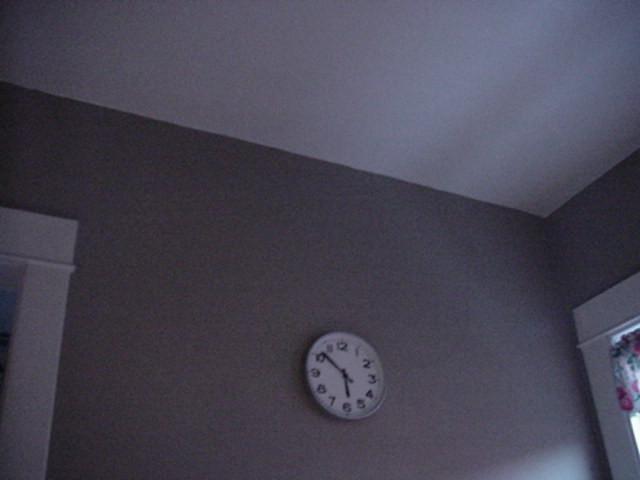The image depicts the upper portion of a somewhat grainy room, featuring a white ceiling and dark gray walls. On the right side of the image, a window allows natural sunlight to stream into the room, indicating that it is daytime. This window is adorned with floral-patterned blinds in green and pink hues. Prominently displayed on the wall is a white-faced clock with black hands. The hands of the clock are positioned precisely, pointing at 5:51. The scene includes glimpses of two door frames—one on the left and the other on the right—both painted in white, matching the color of the ceiling. The overall ambiance of the room suggests it could be a child's bedroom, lit naturally due to the lack of artificial lighting.